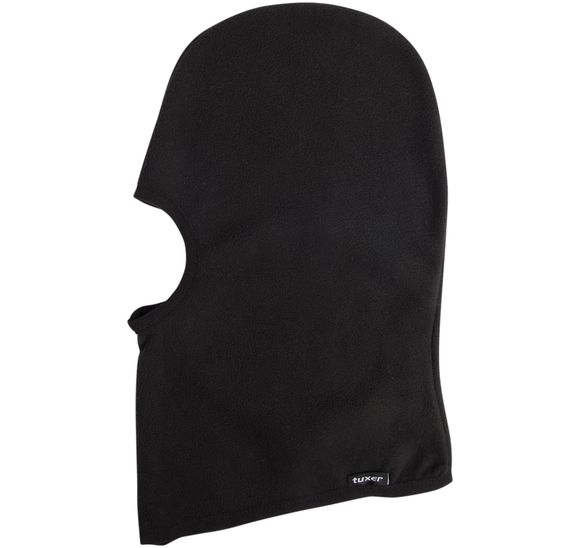The image depicts a neatly folded black balaclava set against a white background, resembling a professional product photo. The balaclava is shown in a side profile view, with the eye opening facing left. The top is rounded, and the bottom edge slopes diagonally upwards from left to right, probably to better fit around the neck. There is a small black tag near the bottom right edge, slightly to the left, with "Tuxer" written in tiny white text. The fabric appears soft and slightly wavy, indicating it's made of felt or a similar material. The overall shape of the balaclava is symmetrical and well defined, making it suitable for a product page on an online store.